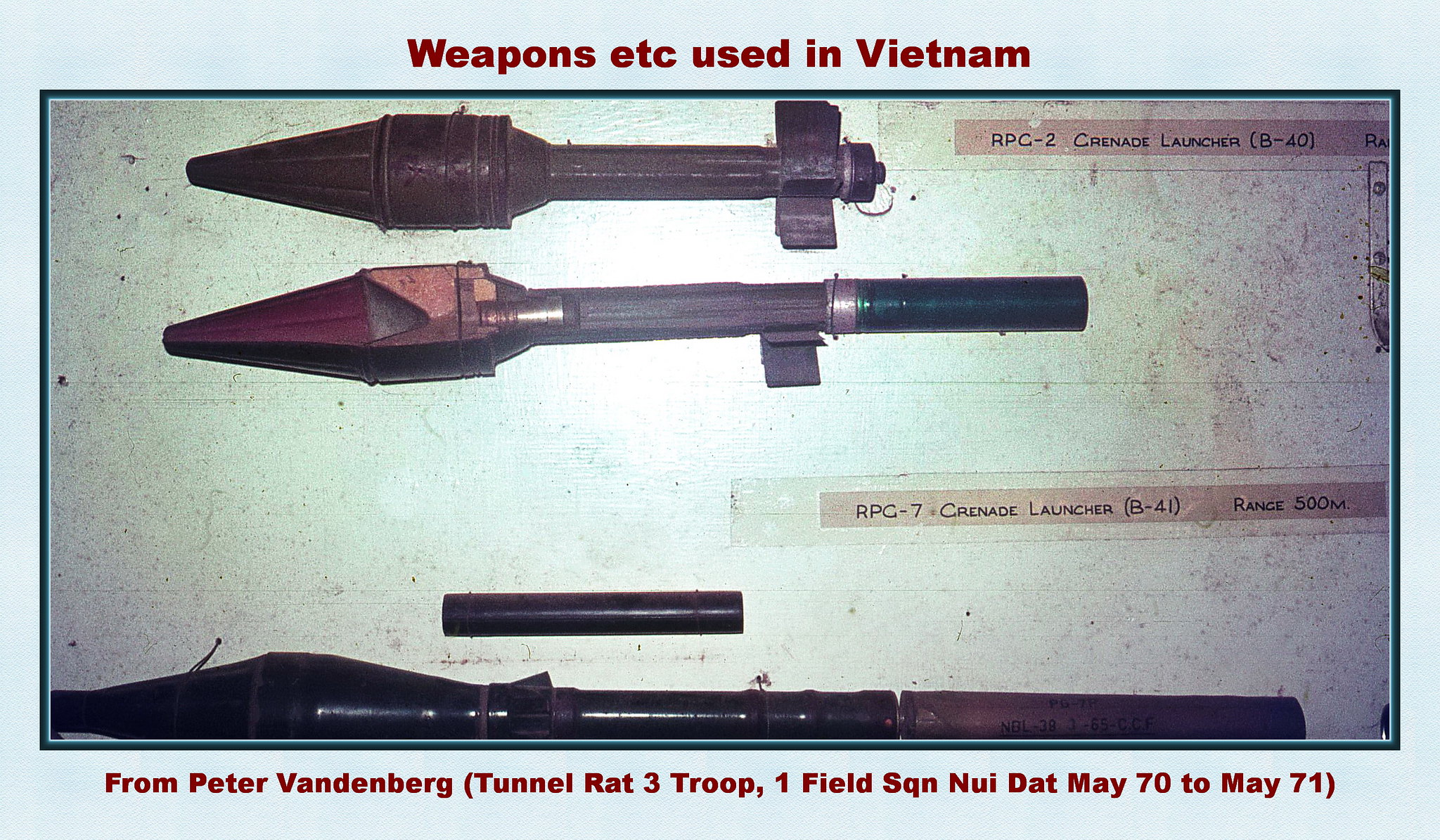The photograph presents a display of historical weapons used in Vietnam, mounted on a light blue backboard. The image has an aged, faded appearance and is framed by a dark blue border. At the top, red text declares, "Weapons, etc. used in Vietnam." Below the photograph, there is an inscription, "From Peter Vandenberg, Tunnel Rat 3 Troop, 1 Field Squadron, Nui Dat, May 1970 - May 1971." The focal point of the display features three different grenade launchers affixed to the board. The first item is labeled "RPG-2 Grenade Launcher B-40," characterized by a conical shape at the top and a long shaft. The second item is similar but lacks a specific label, appearing to be a larger counterpart or an attachment. The third weapon, marked "RPG-7 Grenade Launcher B-41," is noted for its longer range of 500 meters.